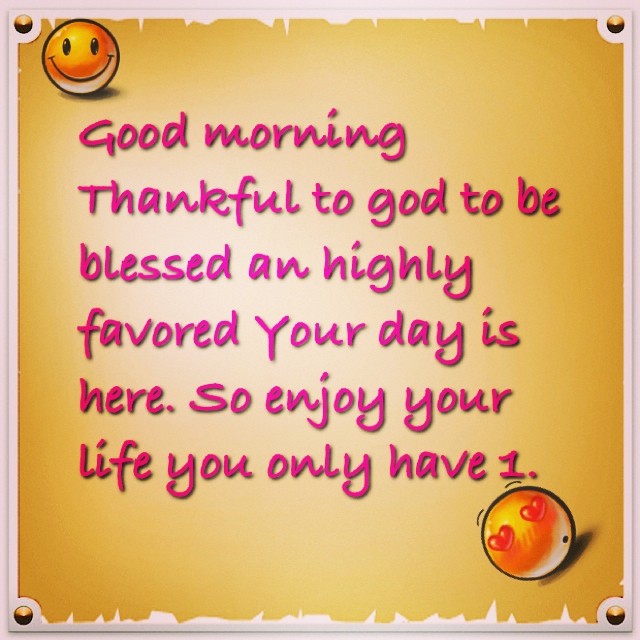The image displays a digitally produced, square-format illustration resembling a motivational social media poster or greeting card. The background appears as a gold-colored, torn parchment paper, lighter towards the center, adding a vintage feel. In the top left corner is a yellow emoji smiley face, while the bottom right features an orange-like emoji with two red heart eyes. Centrally located, the inspirational message in pink script with a black drop shadow reads, "Good morning. Thankful to God to be blessed and highly favored. Your day is here. So enjoy your life. You only have one." The overall design includes brass tack-like accents on the four corners, further enhancing its crafted look. The color scheme prominently features shades of white, tan, yellow, orange, purple, red, and gray.